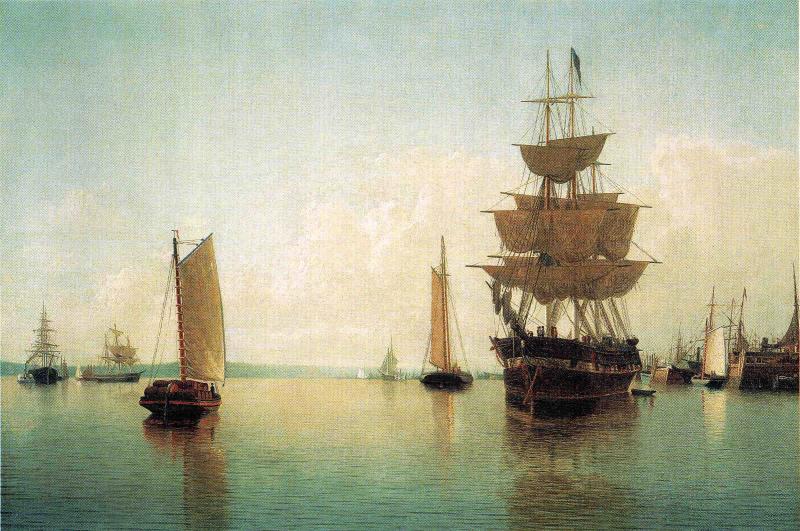This detailed painting depicts a serene maritime scene from a bygone era, showcasing a multitude of vintage wooden ships and boats with cloth sails. In the center of the composition, a large body of calm water reflects the various vessels. The sky above is a gradient of faded blue with white, fluffy clouds, transitioning to a light blue near the horizon and tinged with light orange. In the distance, grayish mountains loom, faint against the sky. On the right side, several boats are docked, their sails lowered, and their masts reaching high into the sky, with one ship prominently featuring half-unfurled sails and a black flag atop its mast. The water beneath shimmers with greenish-yellow reflections of the boats. This margin of the image resembles a dock. The overall ambiance of the painting is tranquil, capturing a moment in time when seafaring life was a common spectacle. The absence of an artist's signature or title suggests the image could be a cropped version or displayed on a web page.